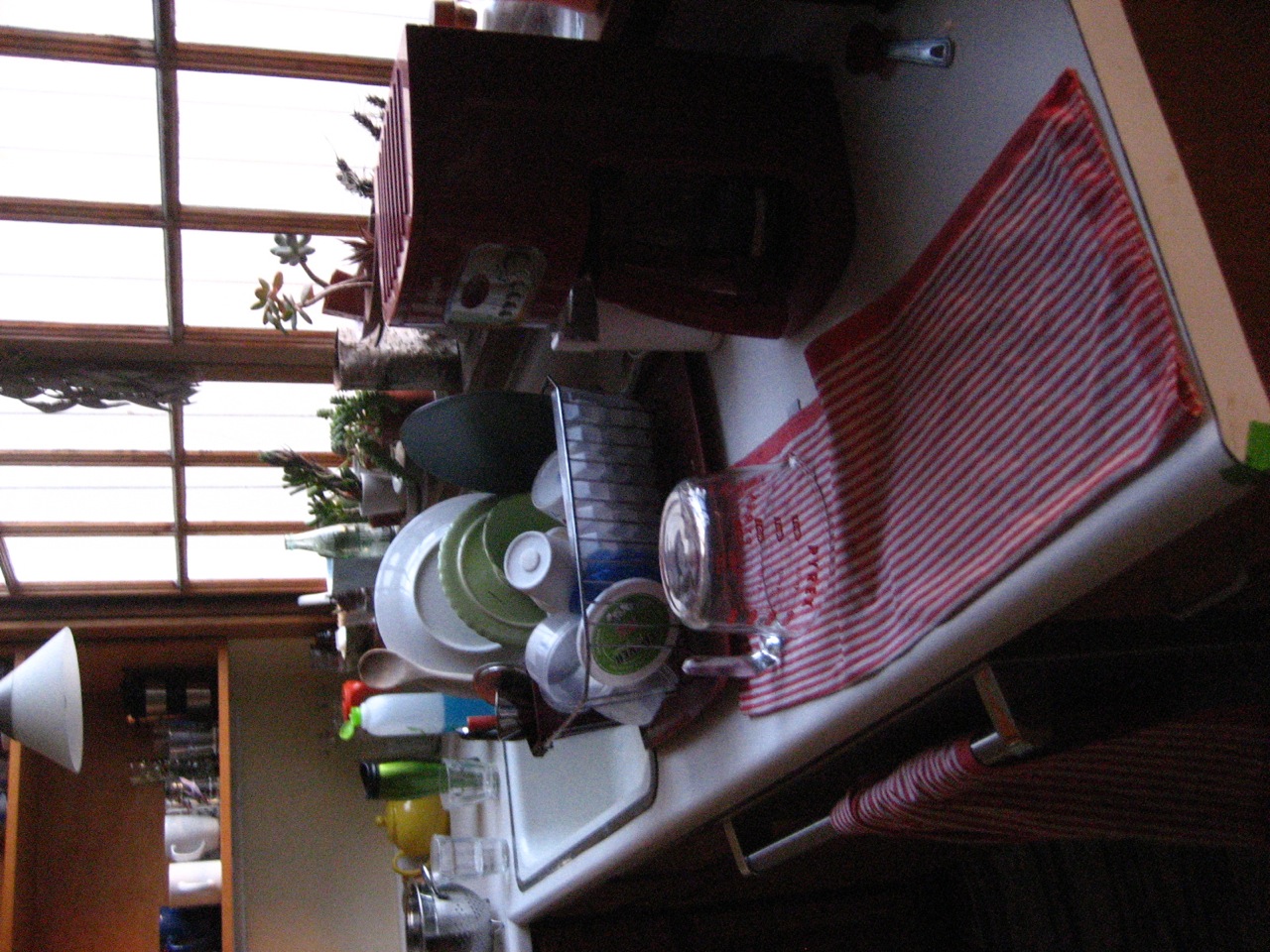The image portrays a cozy kitchen scene with several charming elements. At the very back, open shelving trimmed in wood is prominently featured, possibly merging seamlessly with the white interior or wall behind it. The bottom shelf houses a classic teapot, while the shelf above it displays an assortment of coffee cups and tumblers. A white hanging light fixture adds a touch of elegance to the space. To the right side, a large, multi-paned window allows natural light to flood in.

In the foreground, a light-colored countertop with speckles is the centerpiece, sporting a stainless steel-trimmed white sink. A dish drainer sits beside the sink, filled with dishes, and nearby, a red and white striped towel is laid out with a measuring cup on top of it, suggesting they ran out of space in the drainer. Further adding to the scene's warmth is a mildly darkened area where a coffee pot is discernible. Adding more charm to the setup, another red and white striped towel is draped from the cabinets above. This detailed kitchen scene captures a blend of functionality and homeliness.